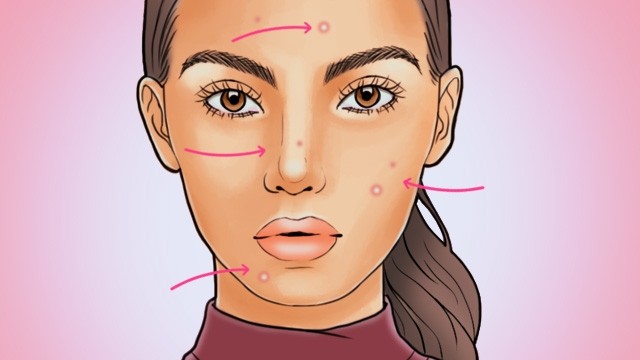This is a close-up image of a detailed illustration of a woman with an olive complexion and notable facial features. She has short, shoulder-length brown hair tied into a ponytail on the right side. Her prominent brown eyes are complemented by symmetrical brown eyebrows and black pupils. The woman’s pink lips exhibit accents of white, and her small ears add to her detailed depiction. She is adorned in a maroon turtleneck, with the illustration cut off just below the collar.

The background of the image is a gradient blend of light pink fading into white. Several pink arrows adorn the woman's face, each pointing to different features and small details. A pink arrow above her left eyebrow points towards a small pink circle on her forehead. Another arrow beneath her left eye directs attention to a pink blotch near her nose, while a pink arrow on her right cheek highlights another pink circle and blotch. Additionally, there is a pink arrow pointing to a small pink dot with a white circle underneath the left side of her chin.

Overall, the image is a rectangular horizontal composition that centers on the animated character with an intricately marked face, set against a faintly blurred pink and white background.